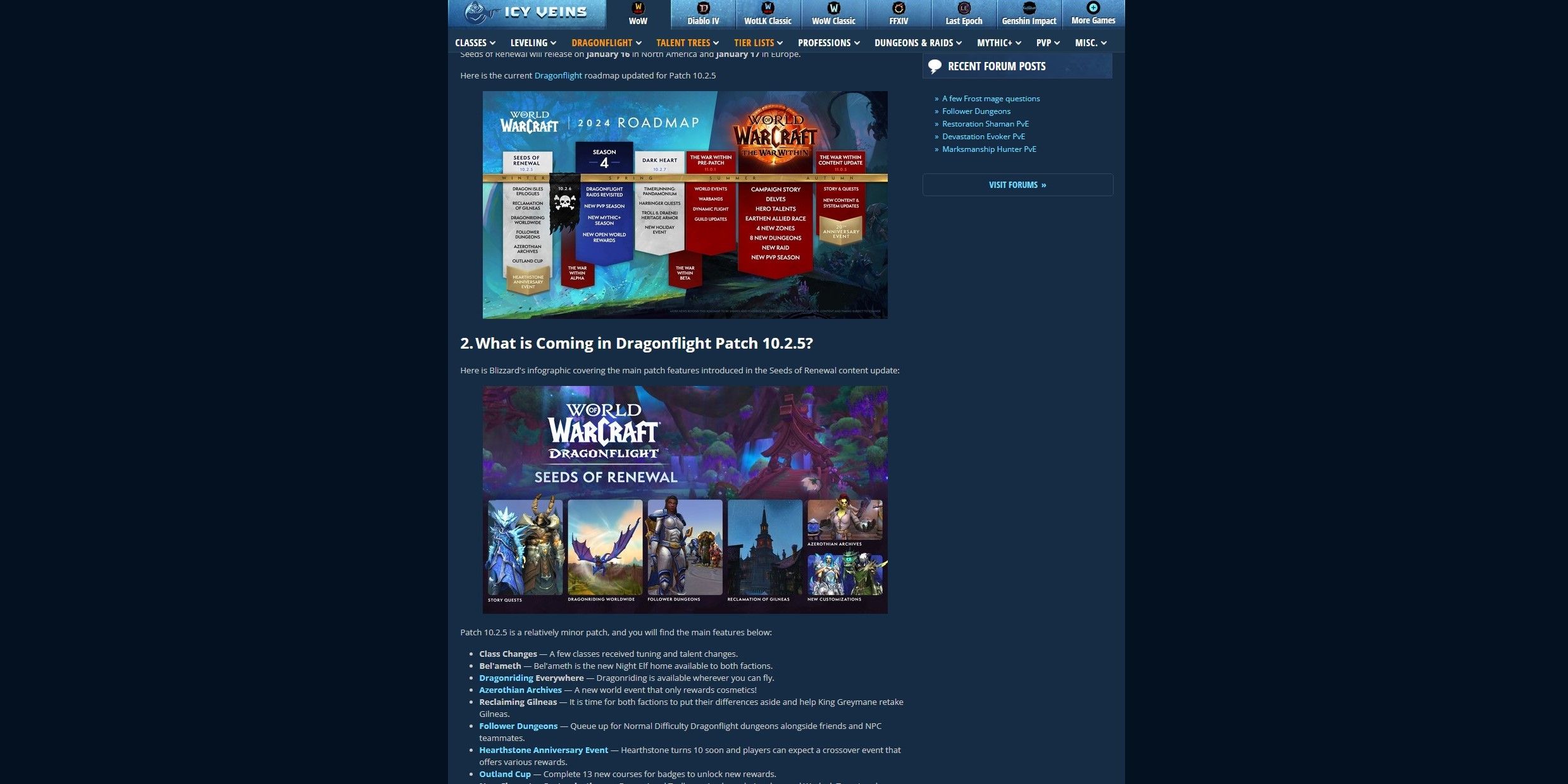This detailed and clean descriptive caption would be suitable for the screenshot:

---

The screenshot captures the main page of the "Icy Veins" website, a popular resource for World of Warcraft news and guides. The page predominantly features two colorful banners.

The first banner, positioned at the top, has a vibrant blue background adorned with vertical stripes in red, blue, and white. At the top of the banner, it reads "World of Warcraft 2024 Roadmap." The first white section on the left is titled "Seeds of Renewal." On the right side, the larger section of the banner is labeled "World of Warcraft: War Within," featuring a glowing sphere. The red banner in this section lists numerous features: "Campaign Story, Delves, Hero Talents, Earthen Allied Force, 4 New Zones, 8 New Dungeons, New Raid, and New PvP Season." A gold band runs horizontally across the banners, marked with tags for "Winter, Spring, Summer, Autumn." Additionally, a black flag with a skull, reading "10.2.4" or "10.2.6," hangs over the far left side of the gold stripe. Below this main banner, there's a line that states "2. What is Coming in Dragonflight Patch 10.2.5."

The second banner beneath displays "World of Warcraft: Dragonflight Seeds of Renewal" and includes five in-game screenshots. The first screenshot shows a story quest with two armored characters. The second is titled "Dragon Worldwide" and features a dragon with purple wings flying in the sky. The third, "Follower Dungeons," also shows armored characters. The fourth screenshot, labeled "Reclamation of Gilneas," depicts a formidable clock tower against a grey backdrop. The fifth and sixth images feature video game characters and are labeled "E010 Archives" and "New Customizations." Below this banner, there is text detailing the patch updates and their specific content.

In the top left corner of the page, a "Recent Post" section from the forum is visible, providing users with up-to-date discussions and information.